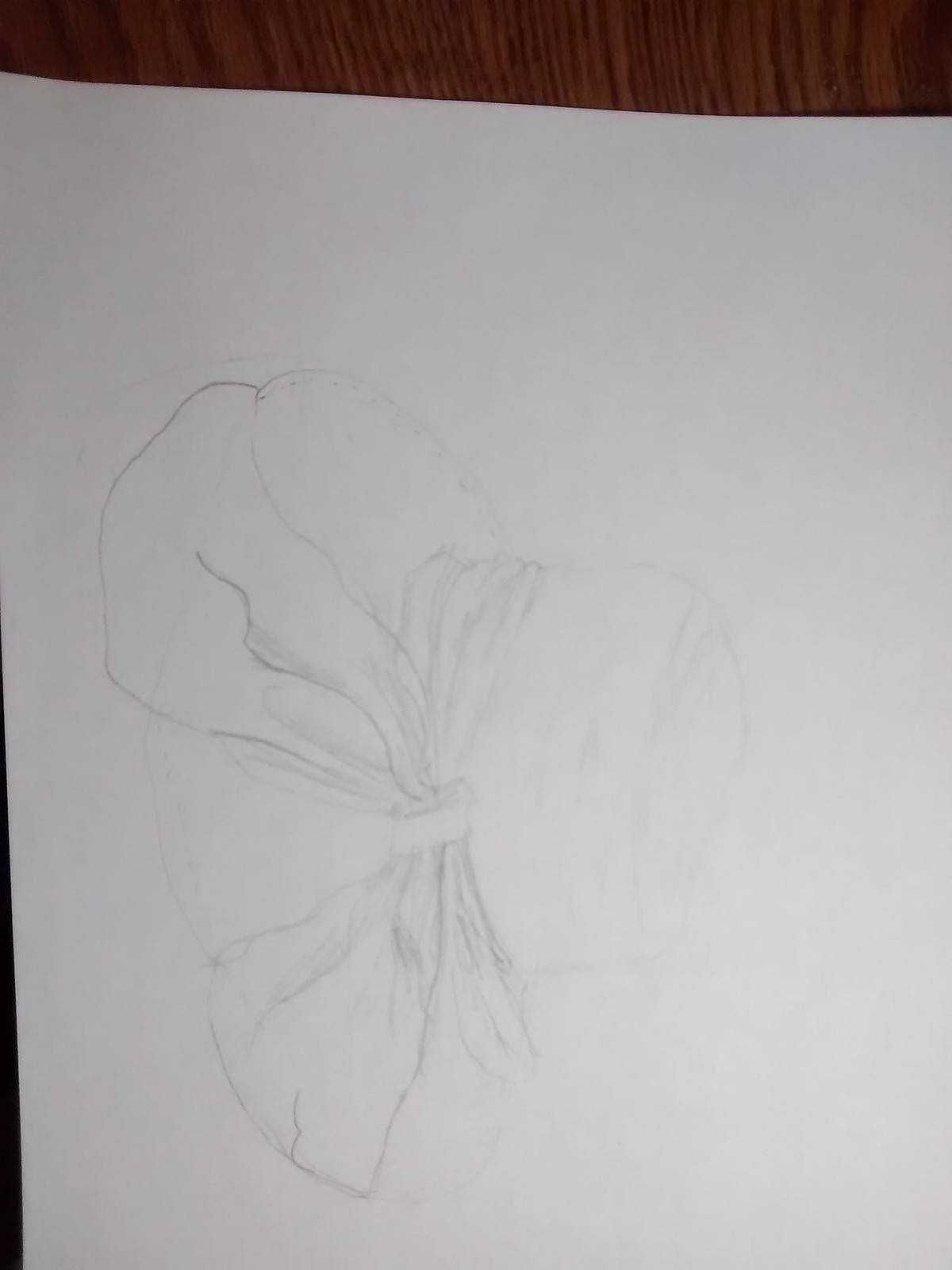In the image, there is a carefully crafted sketch rendered on a sheet of white sketch paper. The paper rests on a dark wood surface, possibly a countertop or desk, which contrasts sharply with the white of the paper. The drawing itself depicts a hat turned on its side, allowing an intricate view of its design. The hat features a rounded brim that encircles the base, with a well-defined crown above it. Adorning the hat is a large, detailed bow that wraps around its structure, partially draping onto the rim. The entire sketch is executed in pencil, showcasing fine lines and shading without any accompanying text.